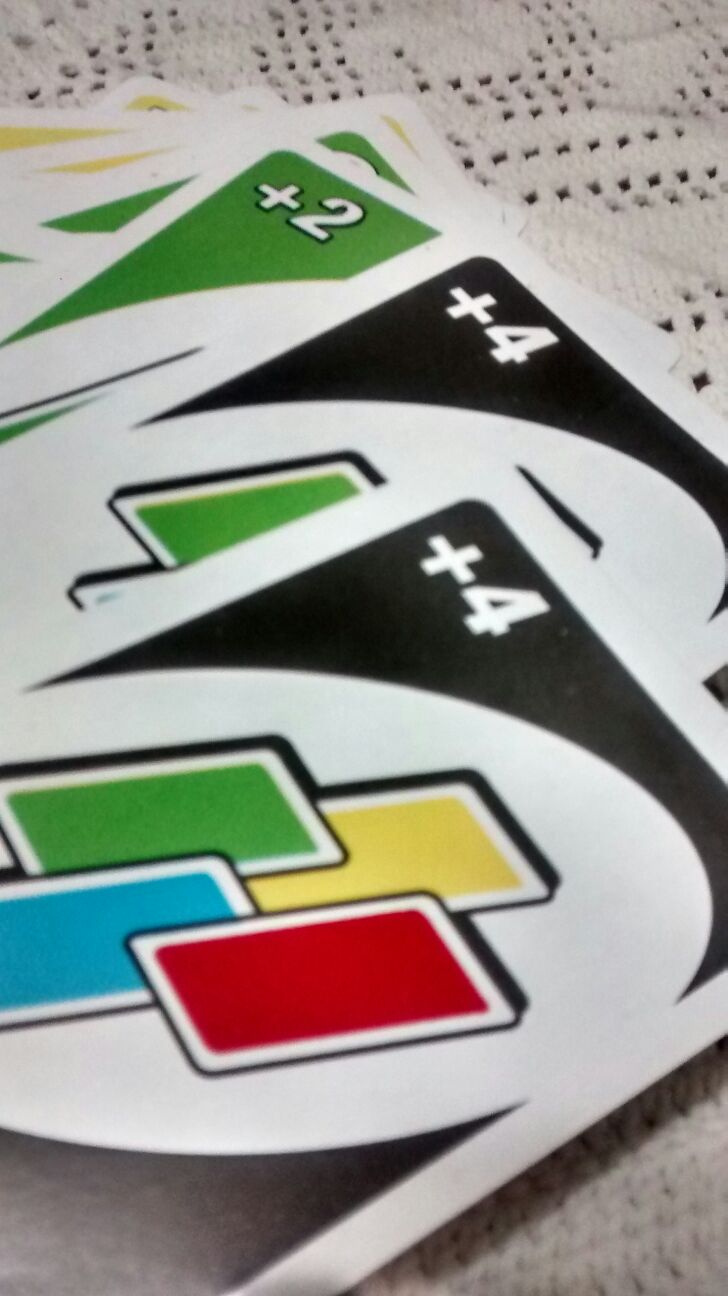This detailed color photograph, oriented in portrait mode, captures a close-up view of UNO cards. The cards are arranged in an overlapping pile and rest on a white crocheted tablecloth with a woven texture. Dominating the forefront of the image are two "wild draw four" cards. These cards feature black backgrounds, white borders, and white ovals in the center. Inside each oval, four smaller, overlapping cards—red, yellow, green, and blue—indicate the draw four action. A plus sign and the number four are prominently displayed in the upper left corner of each card. Behind these, there is a green "draw two" card, identifiable by its green background and the plus two in the upper corner. Further back, a stack of yellow cards is partially visible, although only their edges can be seen. The intricate details, such as the woven tablecloth and the precise arrangement of the cards, highlight the tactile and visual elements of the scene.